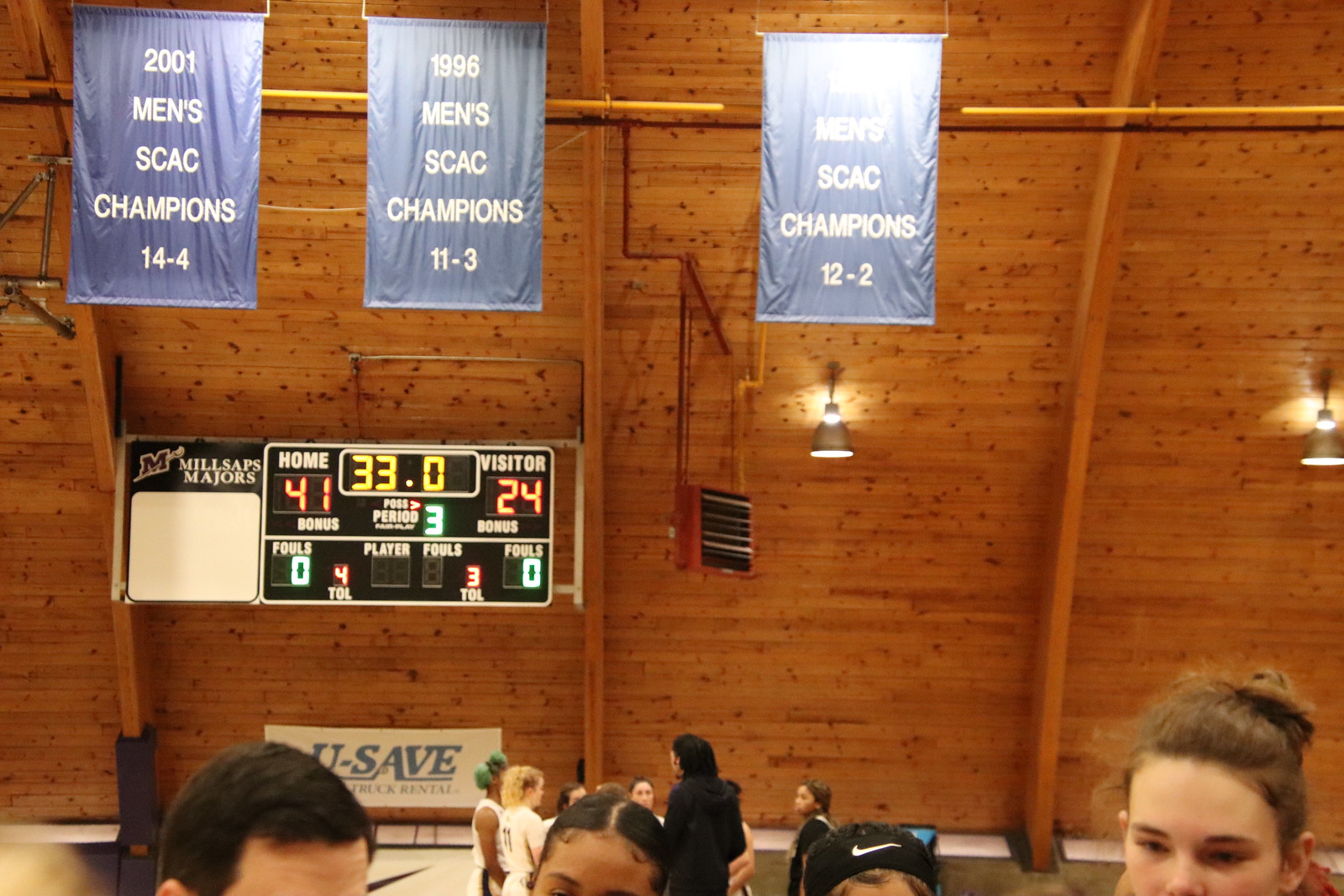The photographic image captures an indoor stadium or arena with a wooden, curved ceiling adorned with hanging spotlights. Three prominent blue banners are suspended from the rafters, commemorating past achievements: "2001 Men's SCAC Champions 14-4," "1996 Men's SCAC Champions 11-3," and another partially obscured banner indicating another championship with "SCAC Champions 12-2." Centrally, a scoreboard reads "Home 41, Visitor 24, 3rd Period, 33.0," with additional details about possession and fouls, flanked by "Millsaps Majors." "USAFE" is also noted on a wall banner. The lower portion of the image shows just the tops of several spectators' heads—including a young man with dark hair, an African-American woman with her hair pulled back, an individual in a baseball cap, and a young white woman with her hair pulled back—while an adult woman in the background converses with younger women in uniform, suggesting a sporting event is underway.